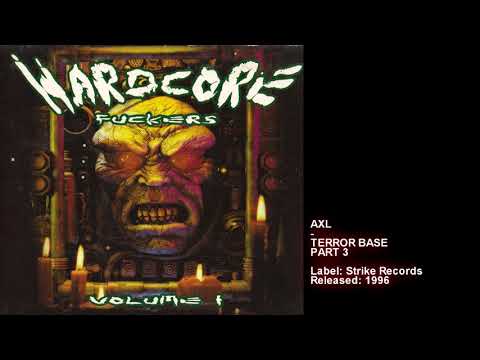The album cover for "Hardcore Fuckers Volume 1" prominently features a grotesque humanoid face with a skin-covered eye area, revealing no eyes. The face, which appears ghoulish and skeletal with decrepit teeth visible in a wide snarl, occupies the central part of the image, framed by a picture frame with four small votive candles—two on each side. The title "Hardcore Fuckers" is displayed in stark white letters with a black outline across the top, emanating an angry vibe, while "Volume 1" is positioned below the face. On the right-hand side of the cover, the text "Axl Terror Bass Part 3" is noted, indicating that it's part of the label Strike Records, and was released in 1996. The entire composition is set against a black background, with the right section of the cover dedicated to the album details.